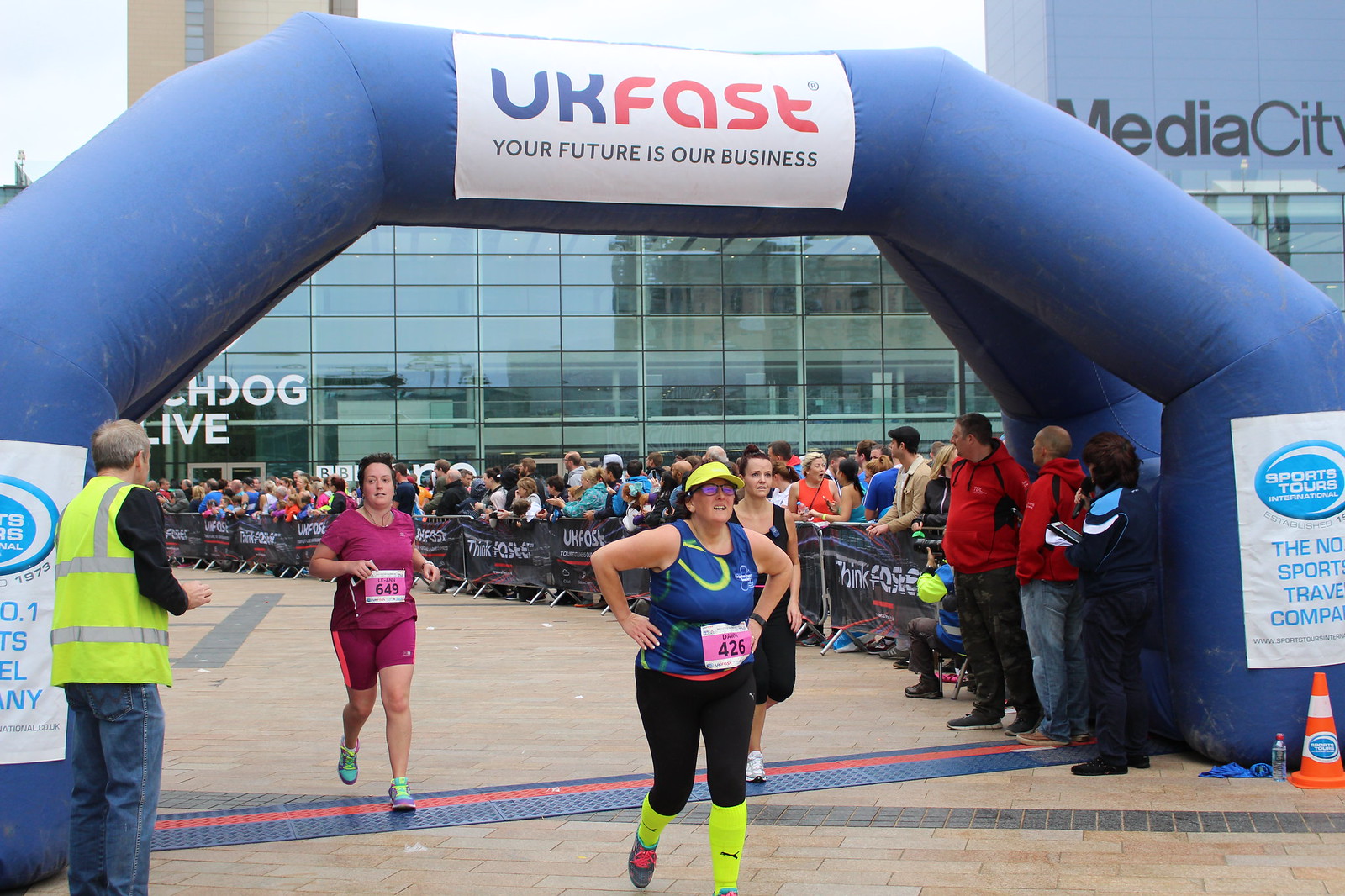This detailed photograph captures the moments at the finish line of a race. In the foreground stands a woman, appearing to be a white female, who has just completed the marathon. She wears a neon green hat, sunglasses, neon green socks, gray shoes with pink shoelaces, and black leggings. Her bluish sleeveless running shirt bears the number 426 on a pink piece of paper at her chest. Her hands are confidently placed on her hips, exuding a sense of accomplishment.

Behind her, to the left, two other runners are visible. The first is another woman, also a white female, wearing a pink outfit with the number 649 prominently displayed. She has blue and yellow shoes, and is crossing the finish line. To her left stands a man in a green safety vest with gray hair; he is facing the runners, seemingly observing the scene. Further to the right of these runners is another woman, dressed in a purple t-shirt and matching purple shorts.

The scene is framed by a blue inflatable arch over the finish line, emblazoned with the words “UK Fast, your future is our business.” Spectators are lined up behind a black banner on the right side of the photo, extending into the background. They stand in front of a tall glass building, adding an urban backdrop to this vibrant and spirited moment.